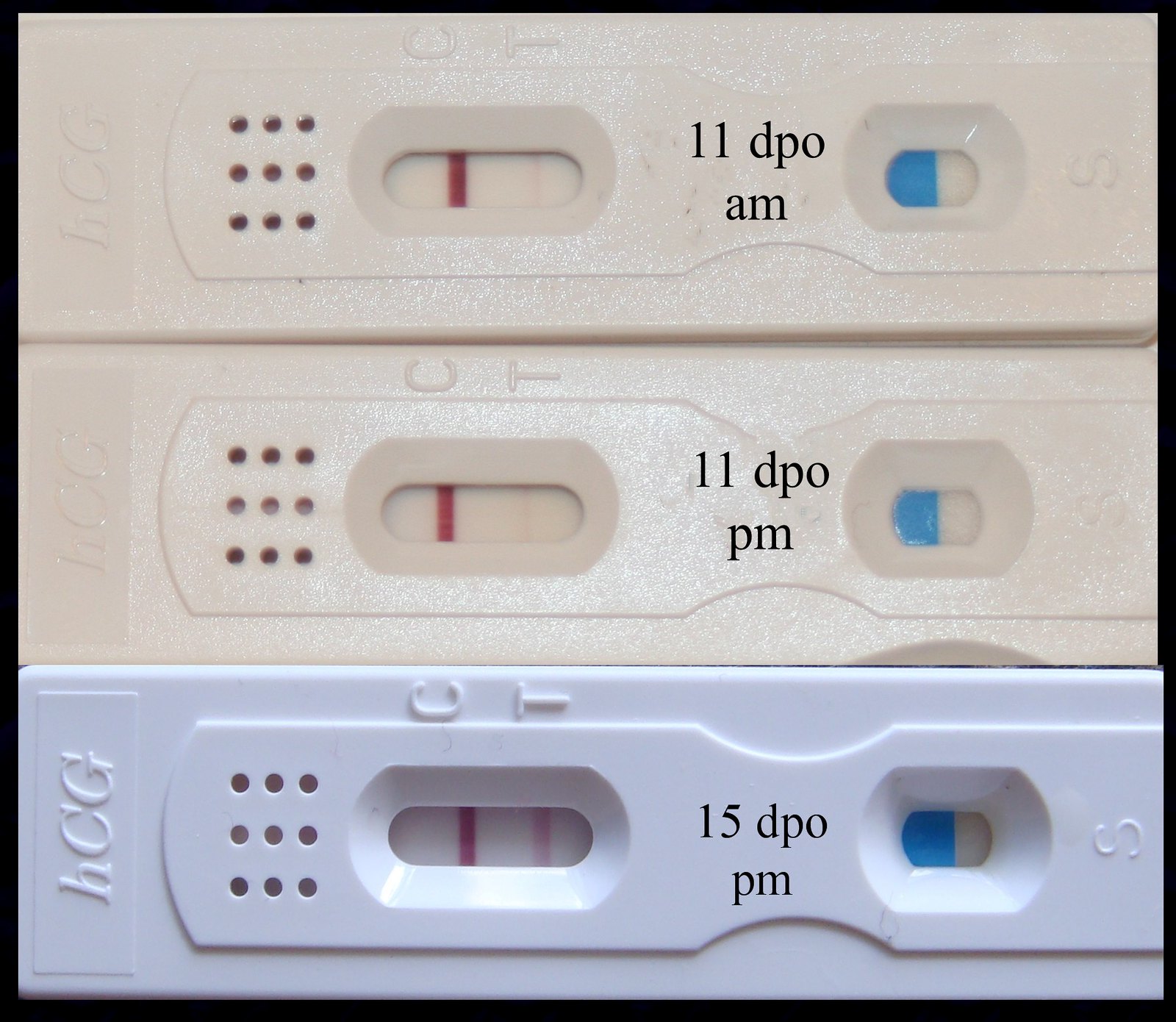The image displays three COVID-19 test kits set against a black border. The bottom test kit, a white device labeled "15 DPO" and "PM," features a solid blue color in the oblong oval section labeled "S." The control line (C) is solid, while the test line (T) is a faint pink. This kit also has nine holes and is marked with "HCG."

The top two test kits are identical, cream-colored, and labeled "11 DPO." Both have a semi-filled blue oblong oval marked "S." Like the first test, the control line (C) is solid, and the test line (T) is faint pink. These kits also feature nine holes and are labeled "HCG." The white kit at the bottom is easier to see compared to the beige ones at the top.